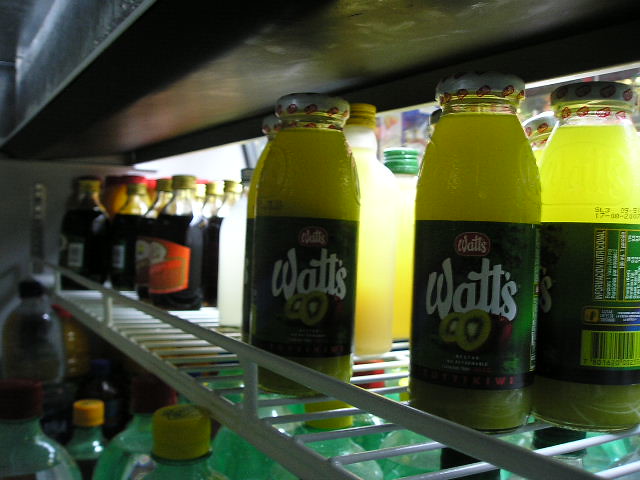This is a detailed close-up photograph of a refrigerated display case, possibly located in a convenience store, grocery outlet, or restaurant. The case prominently features various bottles of beverages. At the forefront on the main white rack, there are several glass bottles filled with a green-yellow liquid labeled "Watts" with images of kiwis beneath the white Watts writing. Some bottles are turned forward, while at least one is turned backward. This middle shelf also showcases other bottles, including clear and green substances with yellow and maroon lids.

In the background, there are more bottles with diverse labels and contents. Notably, there are bottles with dark-colored liquid and distinct orange and brown labels. A lower shelf, partially visible, holds plastic bottles with yellow tops. The structure of the case includes a dark gray and brown industrial-looking top with metal elements that might suggest the underside of a counter. Overall, the photograph captures a well-organized refrigerator shelf brimming with different types of drink bottles, ranging from kiwi juice to potentially soda.